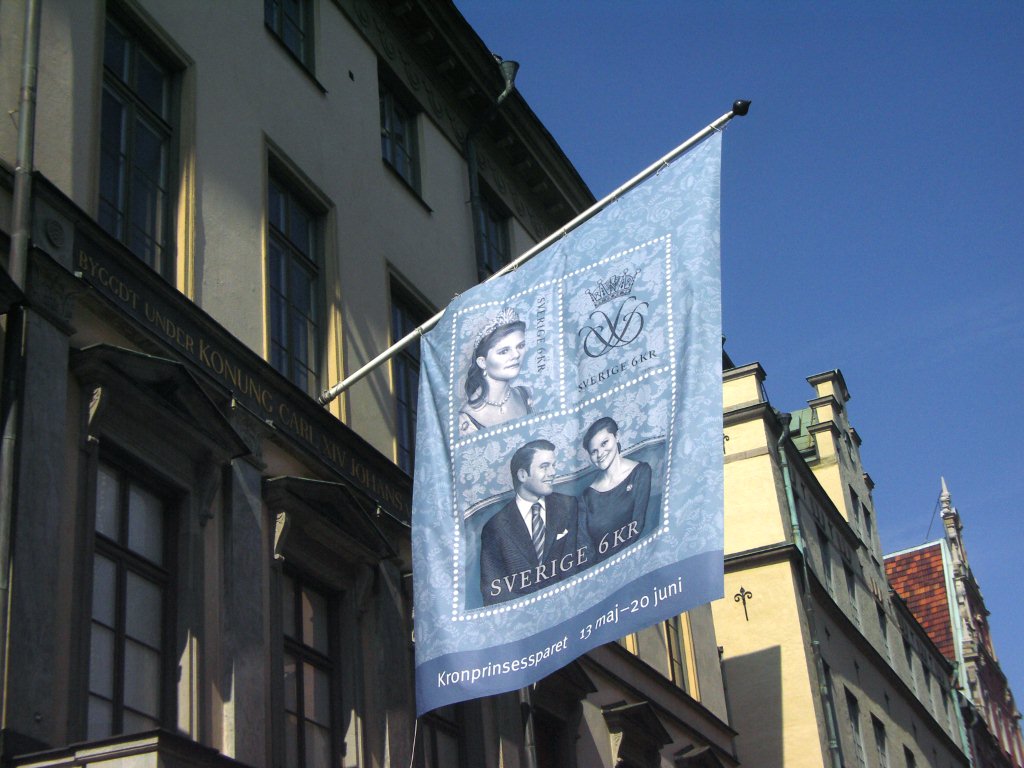The image captures an upward view of an old English or European building, adorned with numerous rectangular windows, under a clear blue sky illuminated by sunlight. Prominently hung on a silver flagpole with a black finial, which extends from between two stories of the building, is a blue flag featuring a detailed floral print background. Central to the flag's design is a series of images bordered by small circular white dots. At the top left, a black and white portrait of a woman wearing a tiara and a necklace, possibly of royalty or a princess, is visible. Adjacent is a logo of interlocking letters topped with a crown, alongside partially obscured text. Below these elements is another black and white image, tinted bluish, depicting a man in a suit with a striped tie and a white pocket square, seated beside a woman in a dark boat neck dress. The man has neatly combed black hair and gazes at the woman, who faces the camera with her hair tied back. The text "SVERIGE 6KR" appears below this scene. At the very bottom of the flag is a blue strip with white fonts reading "Kronprinsessparet 13 Maj - 2021".